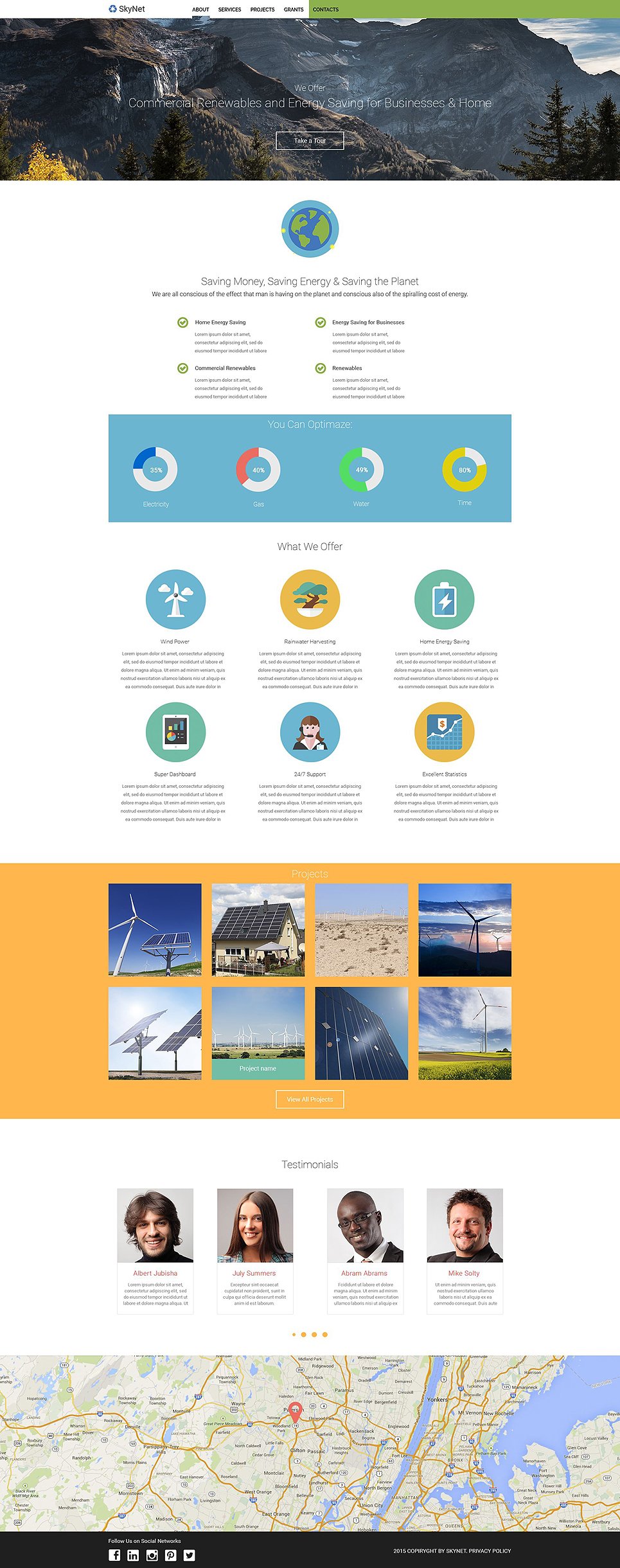In this screenshot, a webpage for the brand Skynet is displayed, focusing on renewable energy and energy savings for businesses and homes. The "About" section is highlighted, providing detailed information on the company’s mission. The slogan "Saving Money, Saving Energy, and Saving the Planet" emphasizes their dedication to sustainable practices. The page showcases various images representing their commitment to renewable energy, including wind turbines, solar panels, and trees. It also features a section with testimonials from four AI-generated individuals, including two white men, a white woman, and a black man, reflecting customer feedback. Additionally, a map with a red pinpoint identifies a specific location related to Skynet's operations or impact.